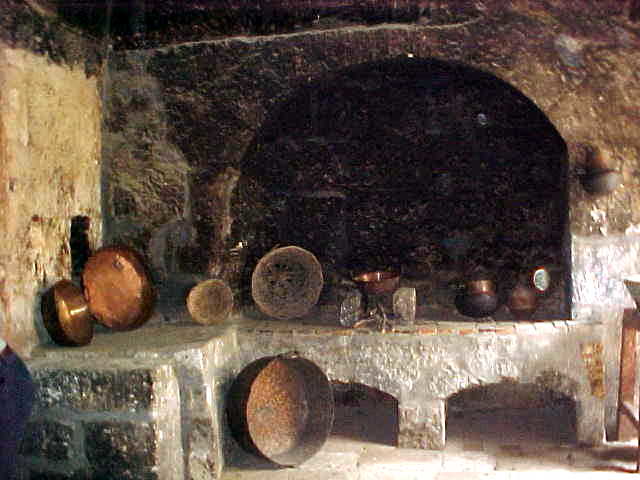The image depicts an ancient, cavern-like kitchen, characterized by its grainy, blurry appearance which suggests it might be either a photograph or a painting. The setting features rocky, grey walls with visible white grouting and a floor that alternates between white and black patches. Central to the scene is an arc-like structure, possibly a historic furnace or stove, surrounded by numerous vessels on a shelf-like structure. A large, round pot is prominently placed sideways in the middle, accompanied by two bricks with sticks in between, supporting a small copper pot, likely part of the stove setup. The overall appearance is aged and dirty, with a lot of soot, indicating it would be laborious to clean. The ancient pottery and the rustic, textured environment give the impression of a long-forgotten place, possibly authentic or perhaps part of a movie set designed to replicate such antiquity.